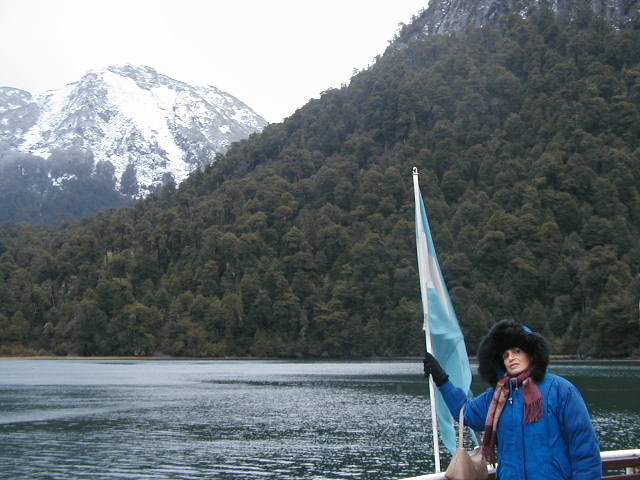The image captures an outdoor setting during the daytime, featuring a Caucasian woman in the lower right-hand corner, posing for the camera. She is dressed in a bright blue winter jacket with a black, fur-lined hood over her head, a red or purplish-toned scarf, black gloves, and holds a pink or cream-colored purse dangling from her right arm. The woman, possibly in her 30s or 40s, has her right arm raised to hold onto a white flagpole with a light baby blue and white flag draped without wind. Behind her, a steel grey, calm body of water extends toward a large hill covered with trees, and in the distance, a snow-capped mountain under a grey-white sky. A metal fence or railing, possibly part of a boat or dock, runs just below her waist, creating a boundary between her and the water.